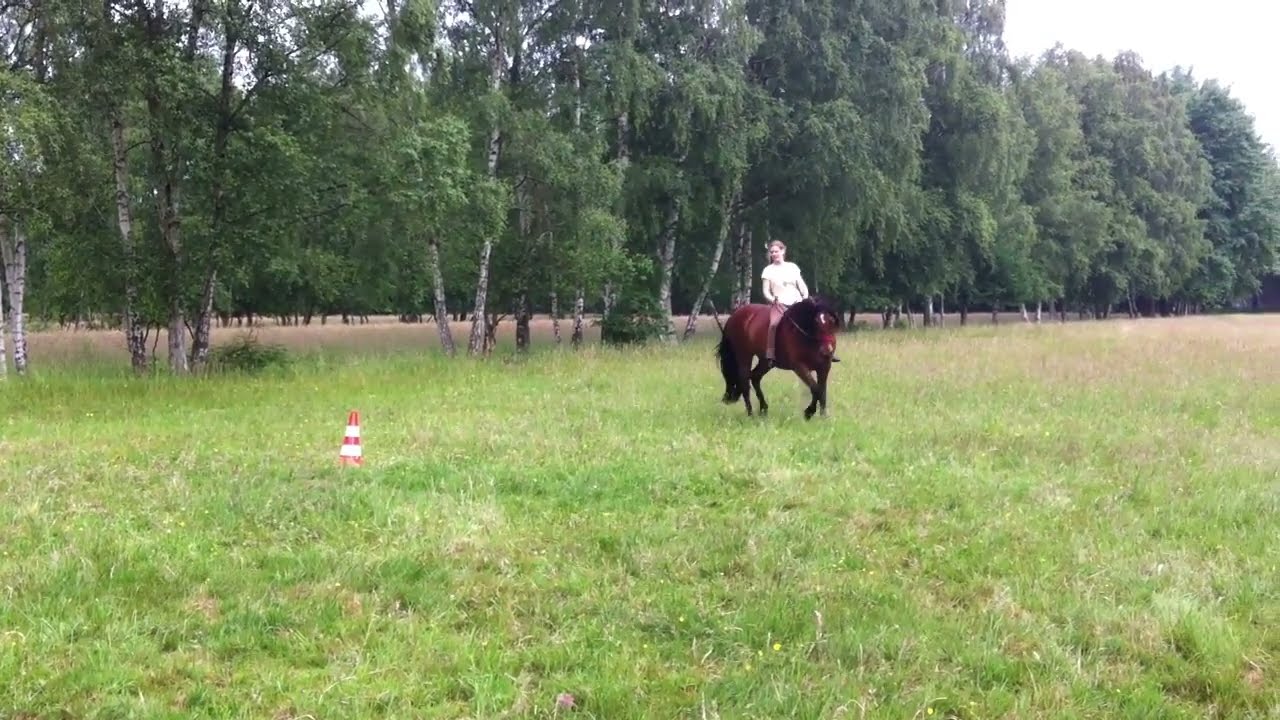In a lush grassland setting with a vibrant green field that turns brownish near the right edge, a man on a brown horse commands the scene. Clad in a white short-sleeved t-shirt, the man rides with confidence as the horse faces forward. Adjacent to them on the left, a red and white striped traffic cone stands out against the verdant background. Behind them, a dense line of tall green trees offers a serene backdrop, with a hinted path weaving through the foliage. The sky remains mostly hidden, creating a somewhat cloudy yet tranquil atmosphere across the landscape.